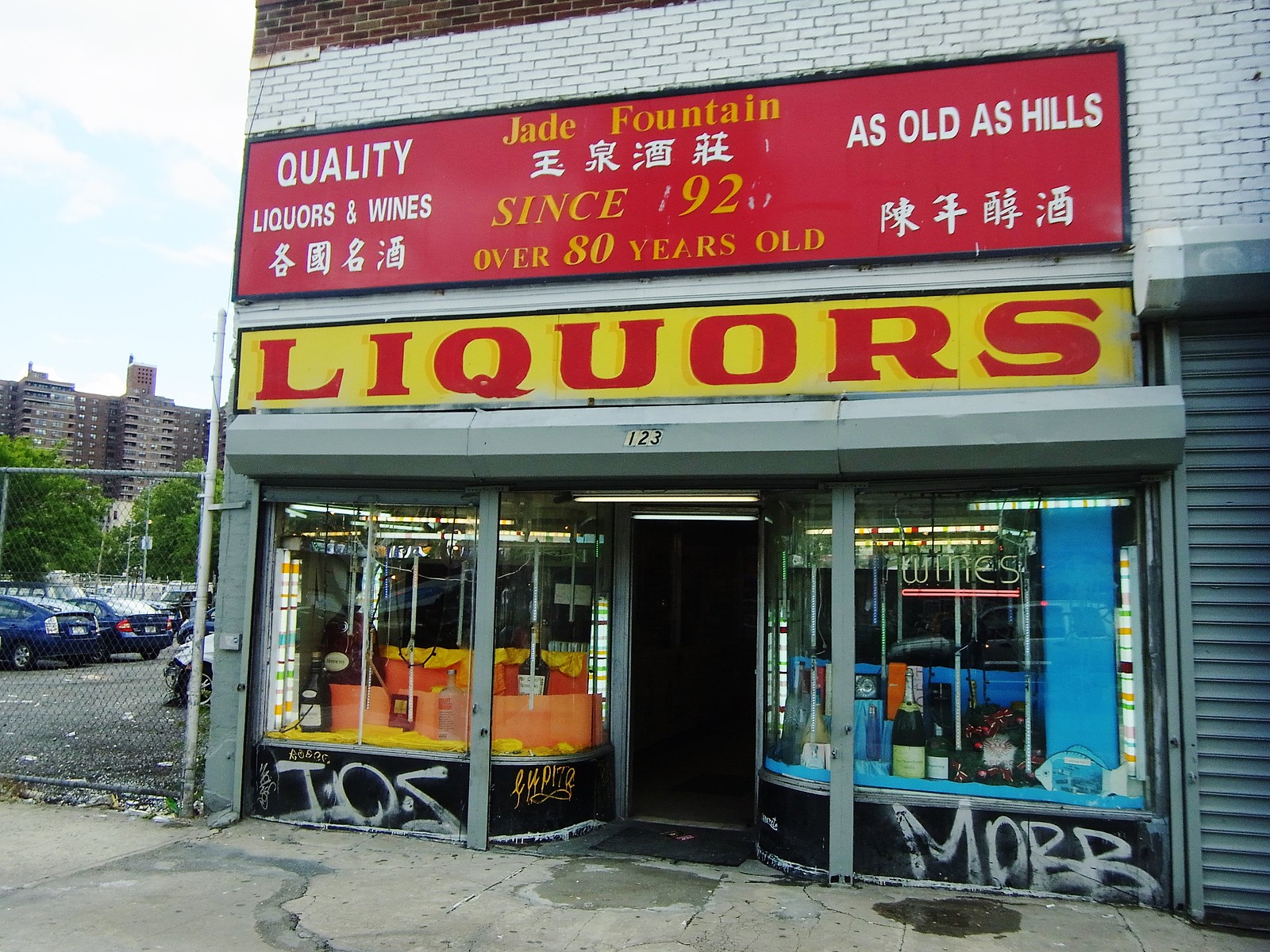The photograph captures the exterior of an old brick liquor store taken during the day, with a cloudy sky overhead. The store, located at the base of an apartment building, prominently features a large, red sign above the entrance that reads "Jade Fountain" in yellow and white letters, accompanied by Chinese symbols and text indicating "Since '92, over 80 years old," and "As old as hills." Adjacent to this is a smaller yellow sign with red letters simply stating "liquors." Below these signs, the store's number "123" is displayed above an open, black door flanked by windows showcasing a decorative display of various blue and orange bottles. A neon sign in one of the windows spells out "wines." The walls beneath the windows are marked with white graffiti, indicating a less well-maintained area. The sidewalk in front of the store is cracked, and there is a chain-link fence enclosing a parking lot beside the building. Beyond the fence, cars and some trees are visible, as well as a large red-brick apartment complex in the background.